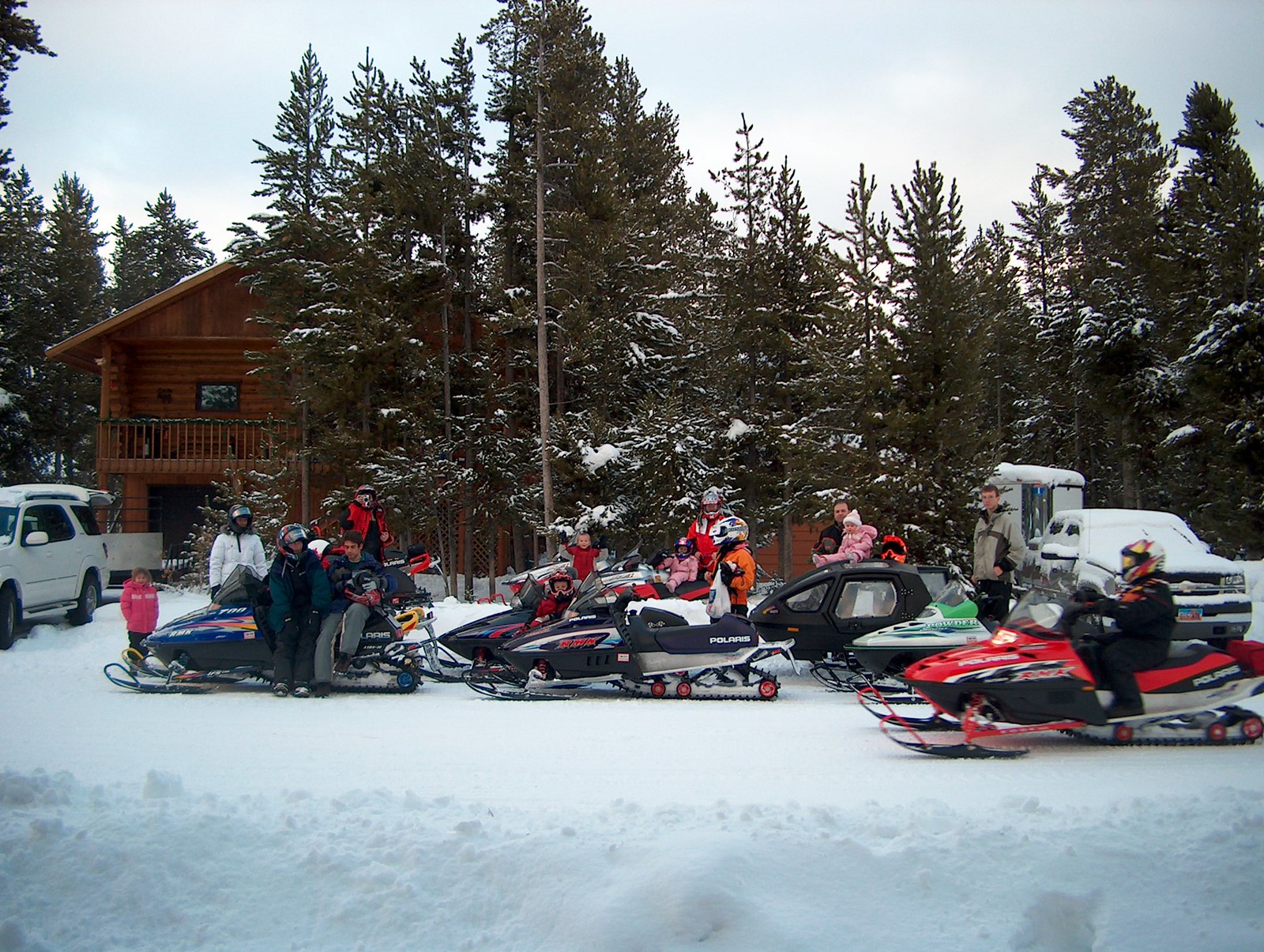The scene is a picturesque winter day outside a rustic log cabin surrounded by tall, snow-covered pine trees. The ground, rooftop, and driveway of the cabin are blanketed in fresh snow. Parked in the lot are seven vibrantly colored snowmobiles, ranging from red to green to black, with some featuring combinations like black with blue or red stripes. Groups of people, all dressed in snowsuits and some donning helmets, are either sitting on the snowmobiles or standing beside them, including a child in a pink snowsuit and a small child being held by an adult. They seem to be posing for a photograph. To the far left, a white SUV with its back hatch open is visible, while on the right side, a Chevy Silverado truck with a thin horse trailer is backed into another driveway. A more snow-covered vehicle, appearing unmoved for a while, adds to the serene, chilly atmosphere of the scene.